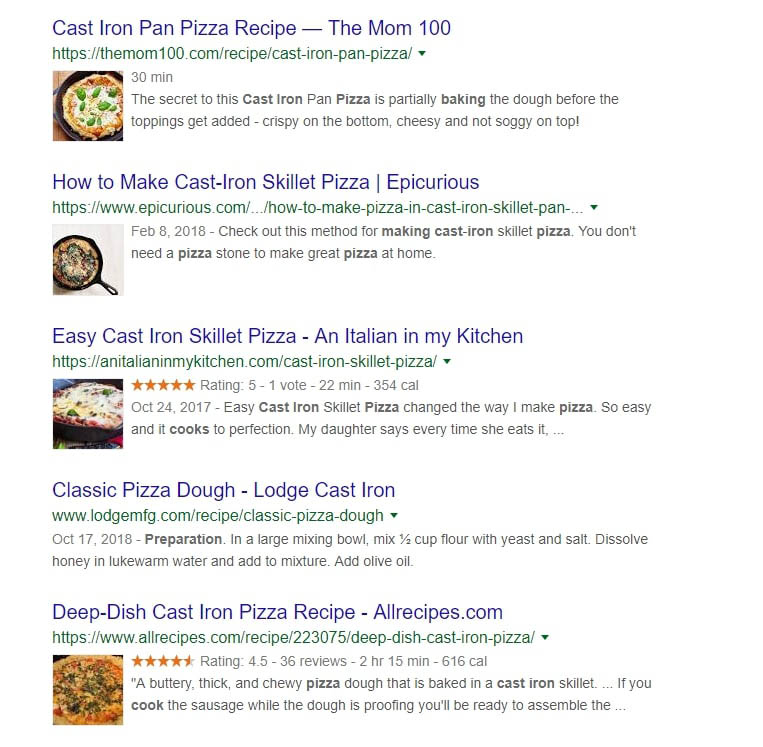This detailed caption was derived from an audio description of a cast iron pan pizza recipe, highlighting the unique method and attributes of cooking pizza in a cast iron skillet, alongside some reviews and personal notes.

---

**Delicious Cast Iron Skillet Pizza Recipe**

Discover the secret to making incredibly crispy and cheesy Cast Iron Pan Pizza from mom100.com. The key to this amazing pizza lies in partially baking the dough before adding the toppings – this technique ensures a perfectly crispy bottom and a delightfully non-soggy top.

**Method Highlights**:
- *Preparation*: No pizza stone required! Use your trusty cast iron skillet for convenience and spectacular results.
- *Dough*: Mix 1 1/2 cups of flour with yeast and salt in a large mixing bowl. Dissolve honey in lukewarm water, then combine with the flour mixture and some olive oil to create a classic pizza dough. Let it proof to achieve that perfect texture.

**Quick Tips**:
- While your dough is proofing, cook your sausage to save time.
- Baking the dough partially before adding cheese and toppings prevents a soggy pizza.

**Reviews & Ratings**:
- Italian in My Kitchen rates this easy skillet pizza 5 stars, highly recommending it as a simple yet delicious meal.
- Allrecipes.com gives it a robust 4.5 stars, praising the buttery, thick, and chewy nature of the pizza dough.

**Background Info**:
- This recipe, featured in multiple cookbooks and highly recommended by home cooks, is known for being an easy and quick dinner option. One reviewer noted that even their daughter's teacher enjoys it!

Enjoy making this deep-dish style pizza with a 22-minute bake time and an estimated 234 calories per serving. Originally posted on October 24, 2017, this method has stood the test of time, continuing to delight pizza lovers everywhere. Happy cooking!